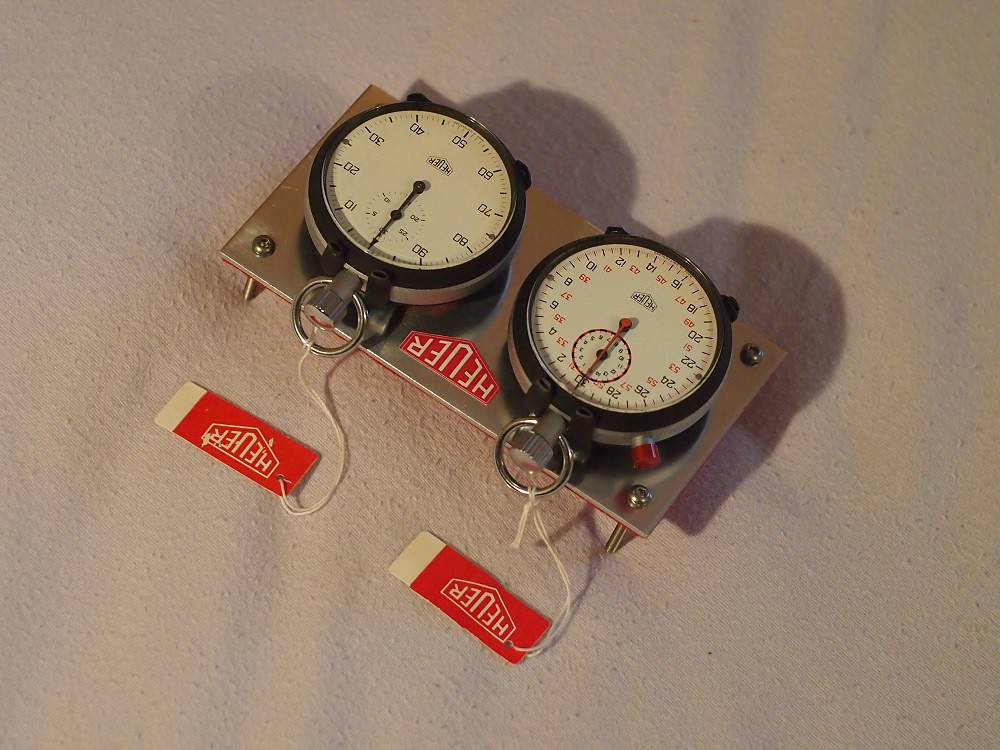This photograph features an upside-down image showcasing two stopwatches mounted onto an off-white, textured wall. The stopwatches are affixed to a stainless steel rectangular sheet that is fastened to the wall. Notably, the mounting screws raise the metal sheet approximately half an inch from the wall, giving it a slightly elevated appearance.

Each stopwatch is circular, framed by a black bezel and backed with silver. The faces of the stopwatches are a crisp white with black numerals and black hands. On the right stopwatch, there is an additional, smaller circle located just below the '12' position, highlighted with red accents. This smaller sub-dial features tiny black numbers and a needle-like red hand. The central part of both stopwatch faces bears a white label inscribed with the word "Hewer."

Both stopwatches also feature circular, silver pull tabs at their tops, from which tags dangle via white strings. The tags are rectangular, predominantly red with white text that reads "Hewer," and the tips of the tags are accented in white. The detailed elements and the precise craftsmanship of both stopwatches are prominently visible against the contrasting wall texture.